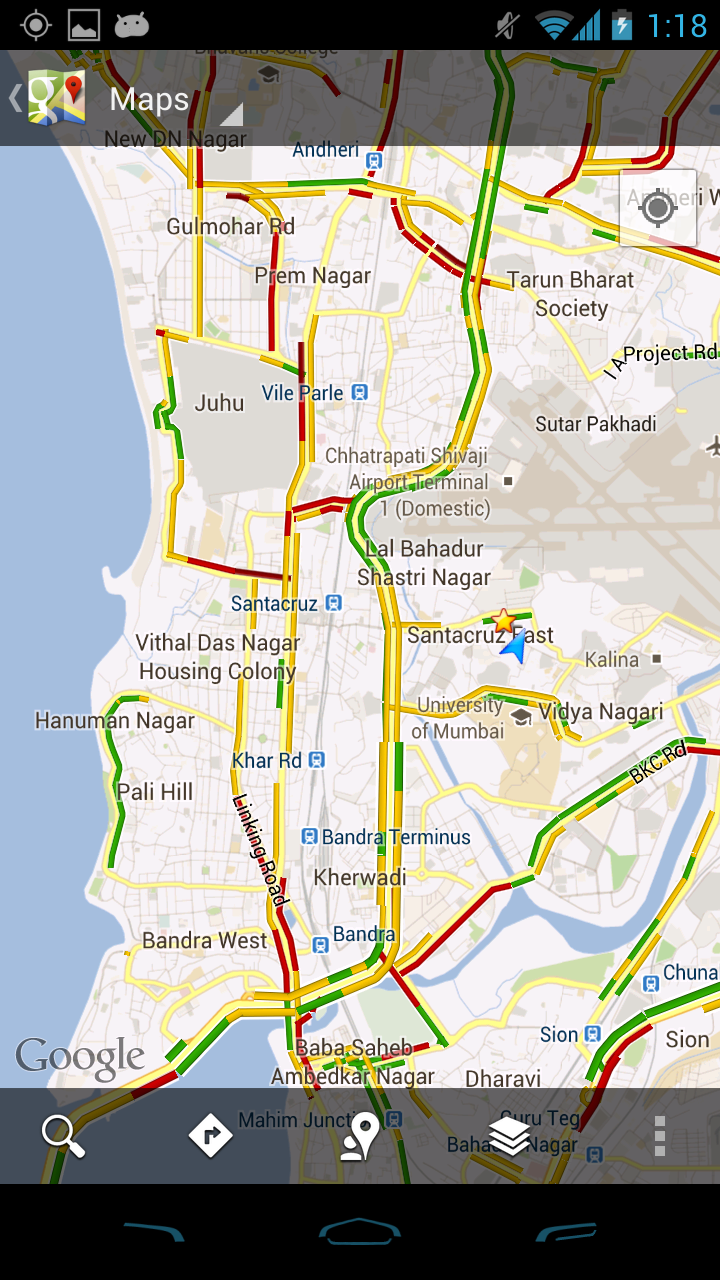This screenshot of a cell phone display features Google Maps open on the screen. The status bar at the top right shows the time as 1:18. The battery indicator displays a usage level between 80% to 85%, the cell phone reception is strong with 4 bars, Wi-Fi is connected with 3 out of 4 bars, and the ringtone is silenced as indicated by the "no sound" icon. Below the status bar, the Google Maps interface is visible. A transparent black bar at the top shows the word "Maps," accompanied by the Google Maps logo to its left. The map itself highlights various locations including Sutarpakadi, Santa Cruz, the University of Mumbai, and Carr Road. The bottom left corner of the map features the word "Google."